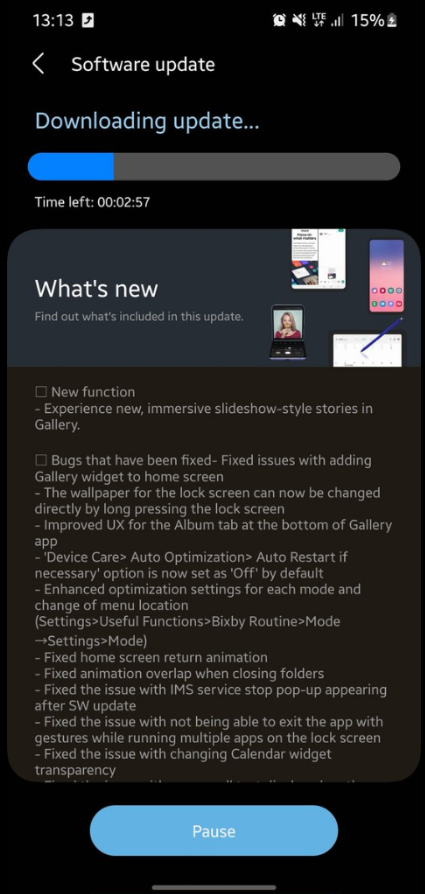The image displays a smartphone screen with a black background. The current time, "13:13," is shown at the top along with a battery level of 15%. An alarm clock icon is present on the screen. Below, the screen indicates a software update process with text in blue reading "Developing or downloading update..." A gray progress bar illustrates about 20% completion. An estimated time left for the update is displayed as "00:02:57."

The screen also details what's included in the software update:
- *New Functions:* Users can now experience new, immersive, slideshow-style stories in the gallery.
- *Bug Fixes:* Issues with adding the gallery widget to the home screen have been resolved. 
- *Improvements:* The lock screen wallpaper can now be changed directly by long pressing the lock screen. User experience (UX) improvements have been made to the album tab at the bottom of the gallery app.

At the bottom of the screen, there's a black rectangle containing a blue oval button labeled "Pause" in white text.